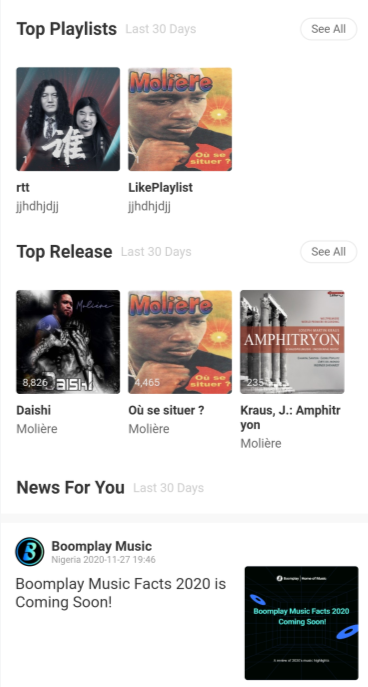This detailed caption describes a screenshot of a music app playlist that is not Spotify:

At the top-left corner, on a white background, the title "Top Playlist" is displayed in black text. Next to it, in very light gray, the phrase "Last 30 Days" can be seen. The playlist includes an image featuring two men with long black hair, and beneath this image, the text "RTT" is visible. The playlist appears to have a nonsensical name, represented by the string "JJHDHJDJJ," which is repeated under the subsequent album cover as well. 

One of the highlighted sections shows an album with the title "Moliere" and features an image of a black man, with the album name printed over his forehead. Below this, there is a category label in black that reads "Top Release," followed by the designation "Last 30 Days." The album in this section lists the artist as "Daishi, Moliere," and while the album titles seem to be in French and difficult to pronounce, they appear to all belong to the same artist or album.

Further down, another category heading in black reads "News For You" with the same "Last 30 Days" timestamp. At the very bottom of the screenshot, there is a profile picture with a gradient from blue to very light green and a bee logo in similar colors. Adjacent to this is the text "Boomplay Music." The caption concludes with the phrase "Boomplay Music Facts 2020 is coming soon."